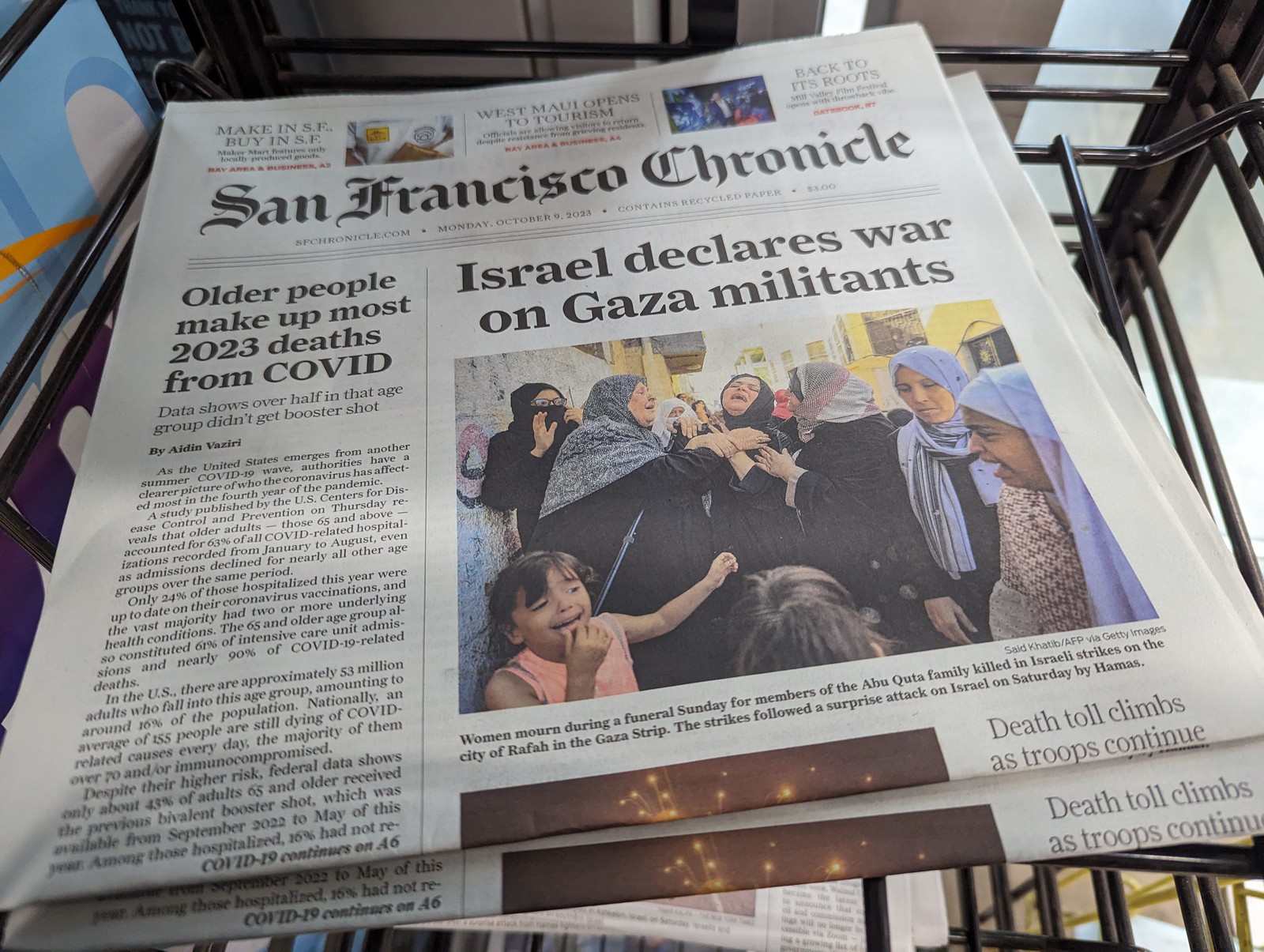In the image, we see a black metal newspaper stand, characterized by its basket-type structure, positioned outdoors with sunlight streaming in. Inside the stand, there are several folded copies of the San Francisco Chronicle neatly stacked. The top newspaper is prominently displayed, with more visible underneath. 

The newspaper's front page features a bold, fancy black font header reading "San Francisco Chronicle." The left-hand column bears the headline in black bold font, "Older People Make Up Most 2023 Deaths from COVID." On the right side, there's a poignant photograph capturing distressed women and a little girl in tears, above which the headline declares, "Israel Declares War on Gaza Militants." Beneath this, partially obscured by the fold, it reads, "Death Toll Climbs as Troops Continue."

The background includes glimpses of an off-white, greenish wall and a gray door, contributing to the sense of an outdoor or semi-outdoor setting. Blue cards are noticeable on the stand's left, enhancing the contextual details. The newspapers themselves have a monochromatic and slightly colored appearance, with hints of blue and pink within the photograph.